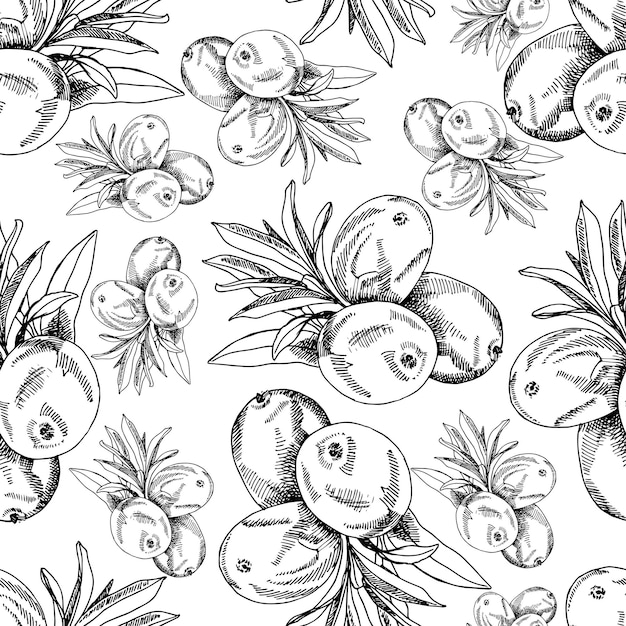This black and white illustration, meticulously rendered in fine pen marks, showcases a dense pattern of fruit clusters. Each cluster, resembling small oval fruits such as olives or berries, contains three fruits. These clusters are repeated throughout the pattern, each one rotated and resized to fill the canvas. Despite the absence of color, the intricate detailing, including spiky leaves and shadowing created by dense line work, gives a vivid depiction of these tropical fruits. The artwork features abundant white space as background, which sharply contrasts with the dark pen illustrations, emphasizing the outlines and depth of the fruits and leaves. This intricate design, with over fifty visible clusters, offers a dynamic visual background that seems almost alive with its constant change in direction and size of the fruit groupings.